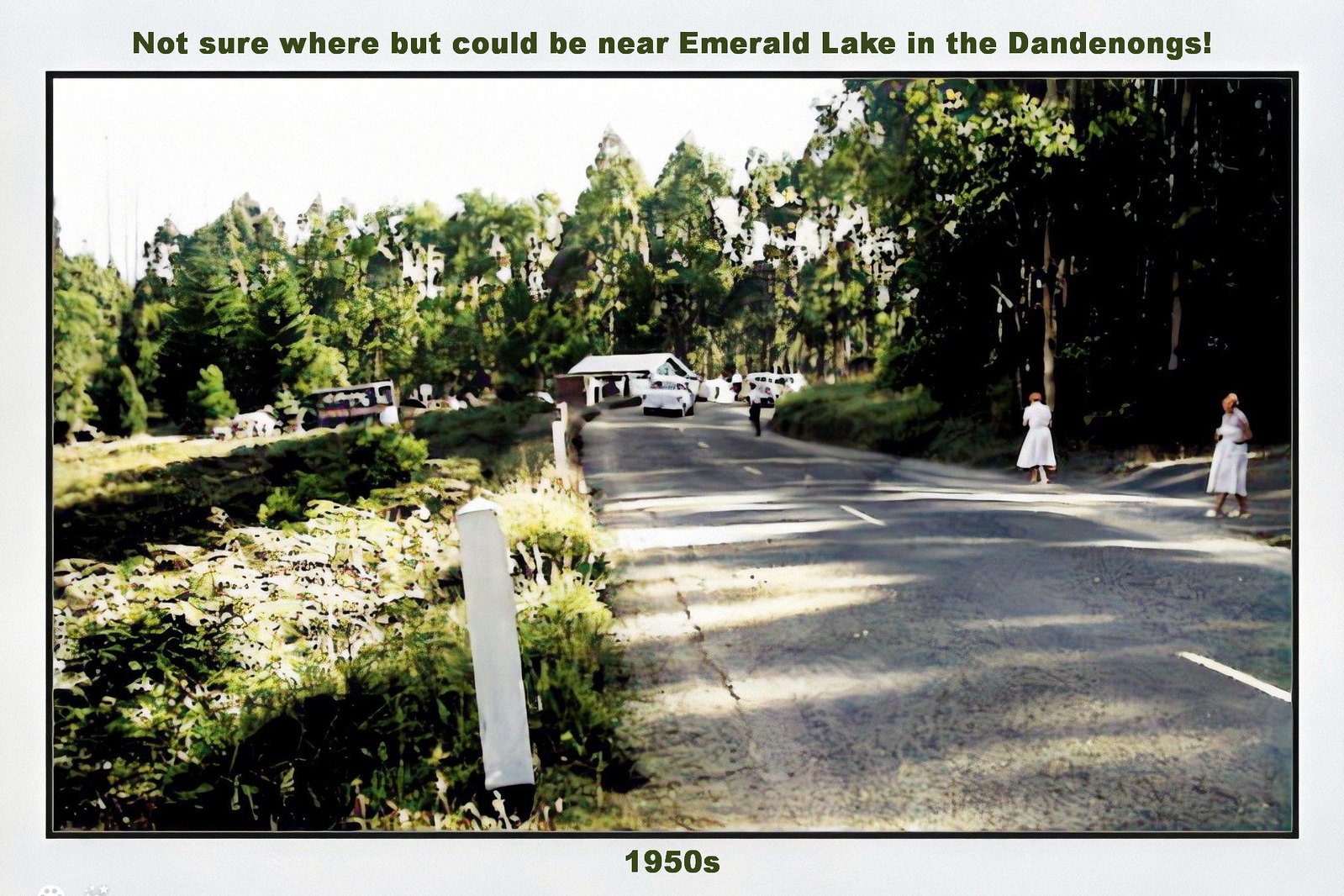The image is an older photograph taken outside on a sunny day, likely from the 1950s, as indicated by the green font beneath the picture. The scene depicts a road starting from the bottom right corner, continuing to the middle, and then curving to the right behind a small hill. Along the right side of the road, two women dressed in white are walking. There is also a gentleman further in the background, dressed in black pants and a white shirt. 

On the left side, the landscape is lush with grass, bushes, and a variety of trees that create a forested backdrop. In the distance, past the curve in the road, there is a small house with several cars parked in front. A dashed white line runs along the middle of the road, guiding vehicles along the path. Close to where the photograph was taken, there is a white post visible in the ground. The image is bordered by text: at the top, in gray-green font, it reads "Not sure where, but could be near Emerald Lake in the Dandenongs," and at the bottom, it states "1950s" in green font.